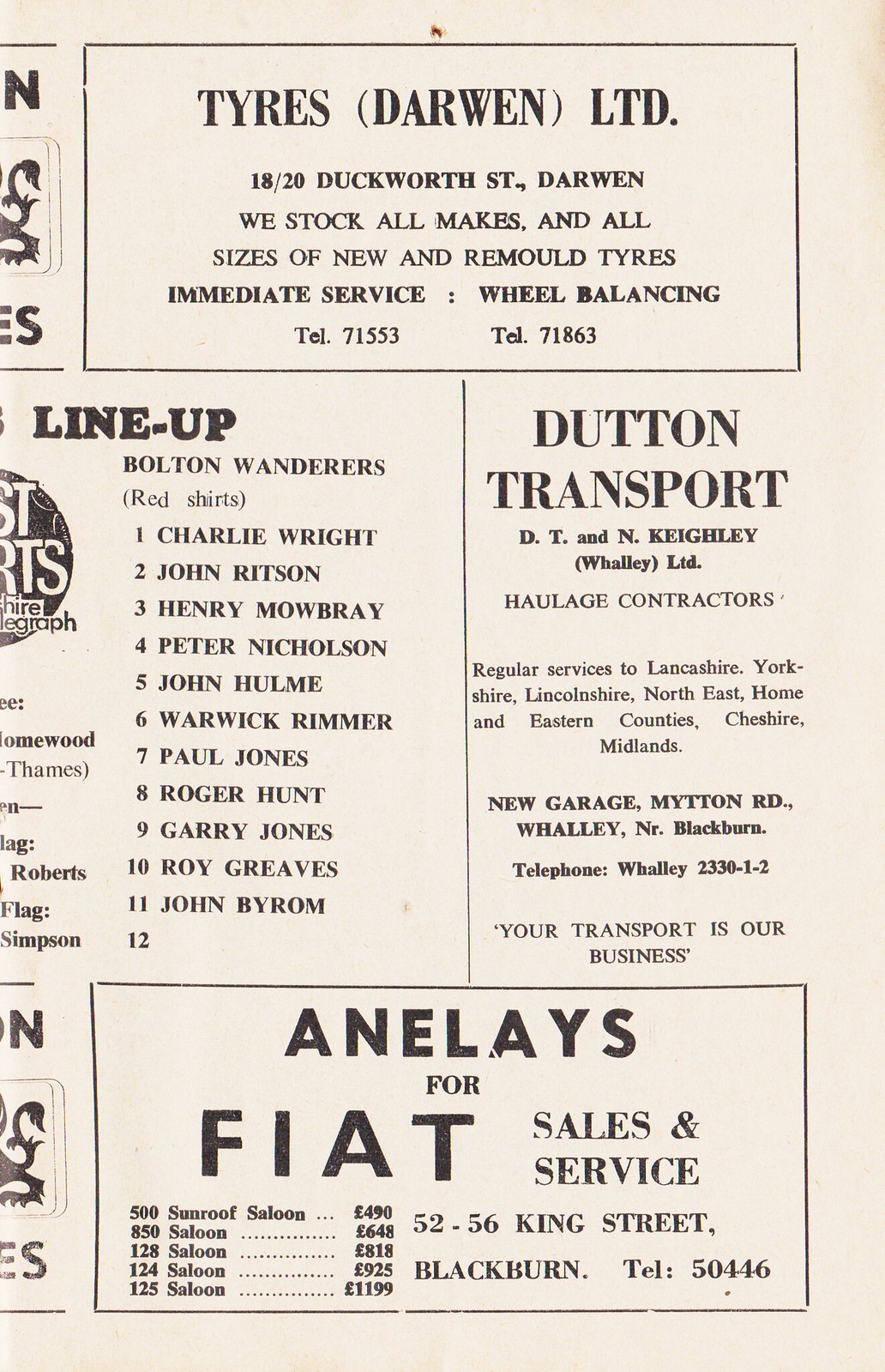The image features a vintage, aged black-and-white printed page from an old sports program or newspaper. Dominating the entirety of the image is a detailed poster, taking up almost all space with its portrait orientation. The paper's background showcases an aged, off-white appearance with browning around the top right corner and a noticeable red stain at the upper center.

At the top of the page, in bold black text, appears an advertisement for "Tires (Darwen) Ltd," providing services like tire stocking of all makes and sizes, immediate service, and wheel balancing, along with their contact information located at 1820 Duckworth Street, Darwen. Below this ad, prominently featured under the bold word "LINEUP," is a roster listing for a sports team with players numbered 1 through 11, likely indicating a soccer or football match lineup.

To the right of the lineup, there is a vertical advertisement for "Dutton Transport, Haulage Contractors," including their contact details and address on Mitten Road, Wally, NR, Blackburn. The bottom of the page contains a horizontal advertisement for "Annalaise" (appearing to be misspelled as Annalyse in one transcription) "Fiat Sales and Service," along with further contact information.

The overall style of the poster is very much vintage, capturing the essence of print publications from a bygone era, with its distinct aged look and minimalistic black-and-white design.